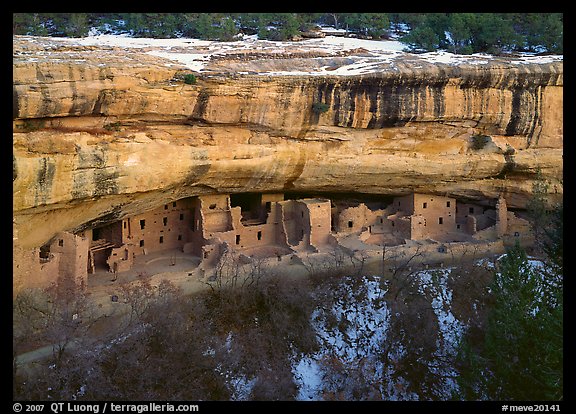The image showcases an ancient heritage site carved directly from a brown-hued hillside, forming the remnants of a historic village or small town that now appears destroyed and eroded. The rocky structures, possibly resembling cabins or small houses, lie beneath a flat-topped mountain partially blanketed in snow and ice, casting an intriguing contrast against the raw, earthen walls. The setting is enriched by a tranquil landscape featuring a nearby small lake that mirrors the surrounding leafless trees and snow. This daytime shot is framed in black, with a watermark in the bottom left corner reading "Copyright 2007, qtleong.com" and another tag on the bottom right corner "#meme20141." The captivating photograph, also identified with terragalleria.com, is an exquisite representation of ancient architecture frozen in time, believed to have survived cataclysmic events or natural upheavals.